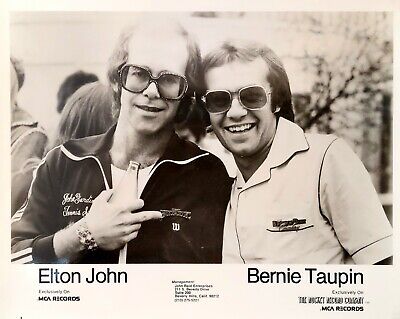This vintage black and white promotional photo captures the legendary duo Elton John and Bernie Taupin during their prime collaboration years. The image, likely distributed by MCA Records, prominently displays the labels "Elton John" and "Bernie Taupin" beneath each man, along with the MCA Records logo. Elton John, with his characteristic flamboyance, sports large, sparkly sunglasses and a zip-up tracksuit jacket layered over a white t-shirt. He’s seen holding a bottle of what appears to be Coca-Cola with his middle finger extended, possibly an unintentional gesture. His balding head is framed by medium-length hair at the sides. Beside him, Bernie Taupin leans in, sharing a bright smile that showcases his teeth. Bernie's attire includes dark sunglasses, a collared shirt with distinctive piping around the edges, and a casual mullet haircut with micro bangs. The background reveals a few blurred heads and tree branches, indicating an outdoor setting. Both artists exude happiness and camaraderie, capturing a moment of their prolific partnership.